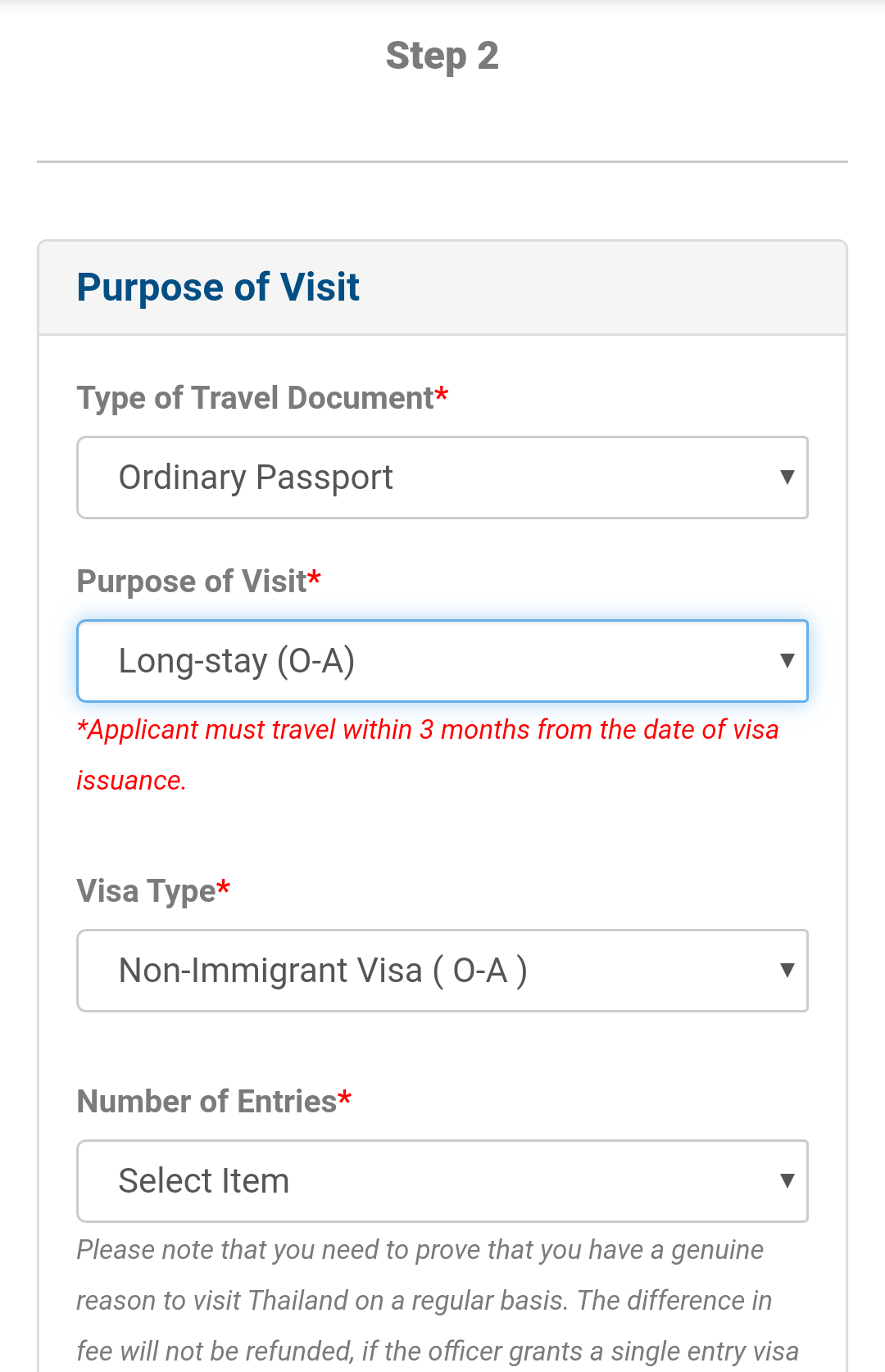This is an image of a screenshot from an application process for a Thai visa, specifically focusing on Step 2: Purpose of Visit. The section begins with the mandatory field "Type of Travel Document," where "Ordinary Passport" is selected. Following that, the "Purpose of Visit" is prompted with a red asterisk, indicating it is a required field, and "Long Stay - O.A." has been chosen. 

Highlighted in red is a warning notice: "Applicant must travel within 3 months from the date of visa issuance." The next field, also marked with a red asterisk, is "Visa Type," where "Non-immigrant Visa - O.A." is selected. 

Underneath, there's a dropdown menu labeled "Number of Entries," which allows the applicant to select the number of times they will enter Thailand on this visa. Below this, there is a note in grey font advising applicants that they must demonstrate a legitimate reason for regular visits to Thailand. Additionally, it states that if the officer decides to grant only a single entry visa, any difference in the fee will not be refunded.